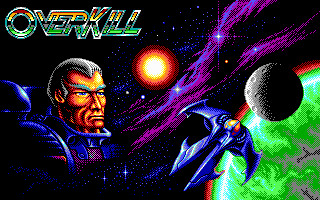This detailed screenshot captures the nostalgic essence of the vintage video game "Overkill." Central to the image are battling spaceships of various intricate designs, each engaging in combat. In the lower right corner, a distinctly alien spacecraft is visible, adding to the diversity of the fleet. Dominating the bottom center is another uniquely designed spaceship, poised for action. On the middle right side, planets drift against the backdrop, enhancing the cosmic setting. The left side features a prominently displayed alien figure with humanoid facial characteristics—slightly elongated ears and distinctive hair—clad in a helmetless spacesuit, embodying a sense of interstellar adventure. The background is a vibrant tapestry of multicolored space gases, with a radiant sun or solar flare situated at the center, casting an ethereal glow. The game's title, "Overkill," is emblazoned in striking green and yellow in the upper left corner, set against a dark backdrop, perfectly highlighting the retro aesthetic. The pixelated texture of the image further evokes the charm of an older generation of video games, contrasting sharply with the high-resolution graphics seen in modern titles.